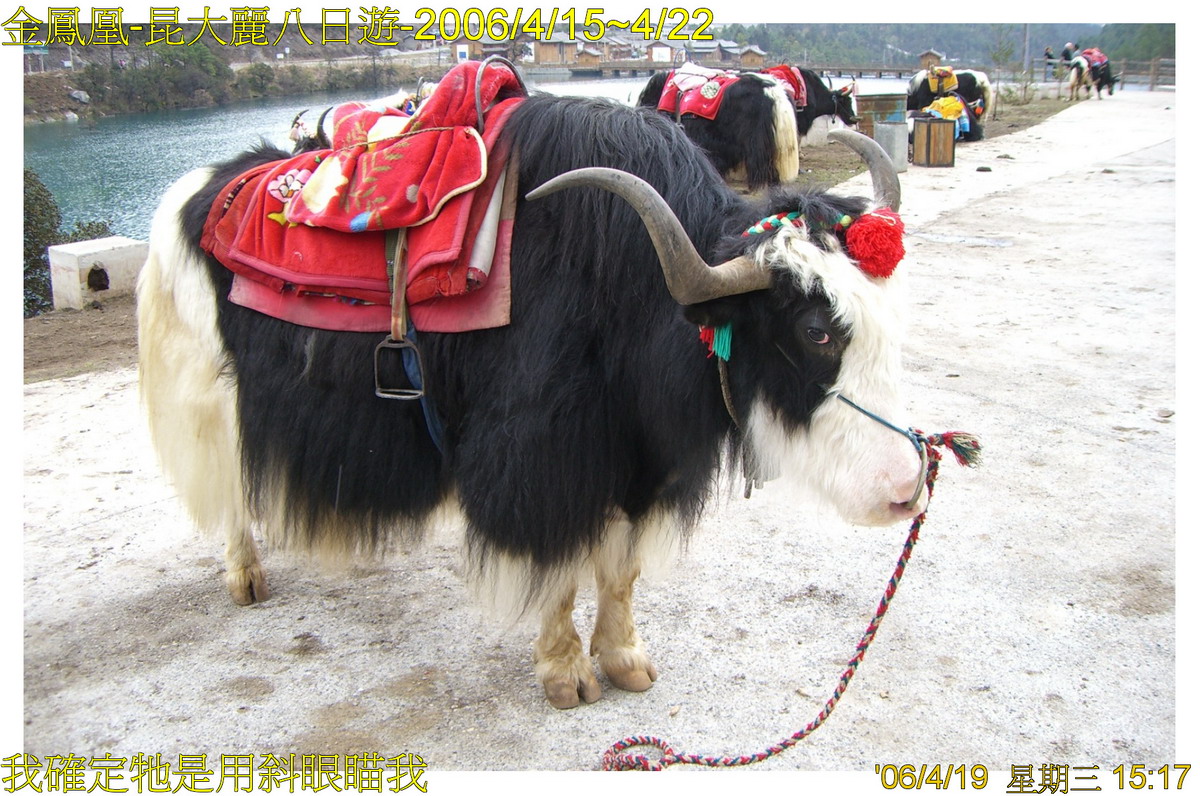This photo captures a scene with several woolly yaks, likely in a region such as Nepal, Tibet, or Mongolia. The main yak in the foreground features a striking appearance with long, thick fur — jet black across its back and sides, and contrasting snow white fur around its butt, face, and up its forehead. This yak sports large, curved gray horns and a red saddle, indicating it is used for riding. The saddle is detailed with cloth straps, stirrups, and a metal bar. The yak’s head is adorned with a red pom-pom and a braided cord in teal, red, and white, complete with a nose ring attached to a rope for steering.

In the background, several other yaks, similarly black and white, are visible. All wear riding saddles and share the decorative pom-poms and halters. They stand on a white ground, which could be a snowy path or a dirt path lightly dusted with something white. Behind these yaks flows a blue river with slight ripples, adding to the scenic outdoor setting.

Text in yellow, featuring Chinese or Japanese characters, appears at the top left and bottom left of the image. A date, likely 2006, is also visible, suggesting the photo's time frame. The overall vivid detail of the scene captures the traditional and rugged lifestyle associated with yak herding in those regions.